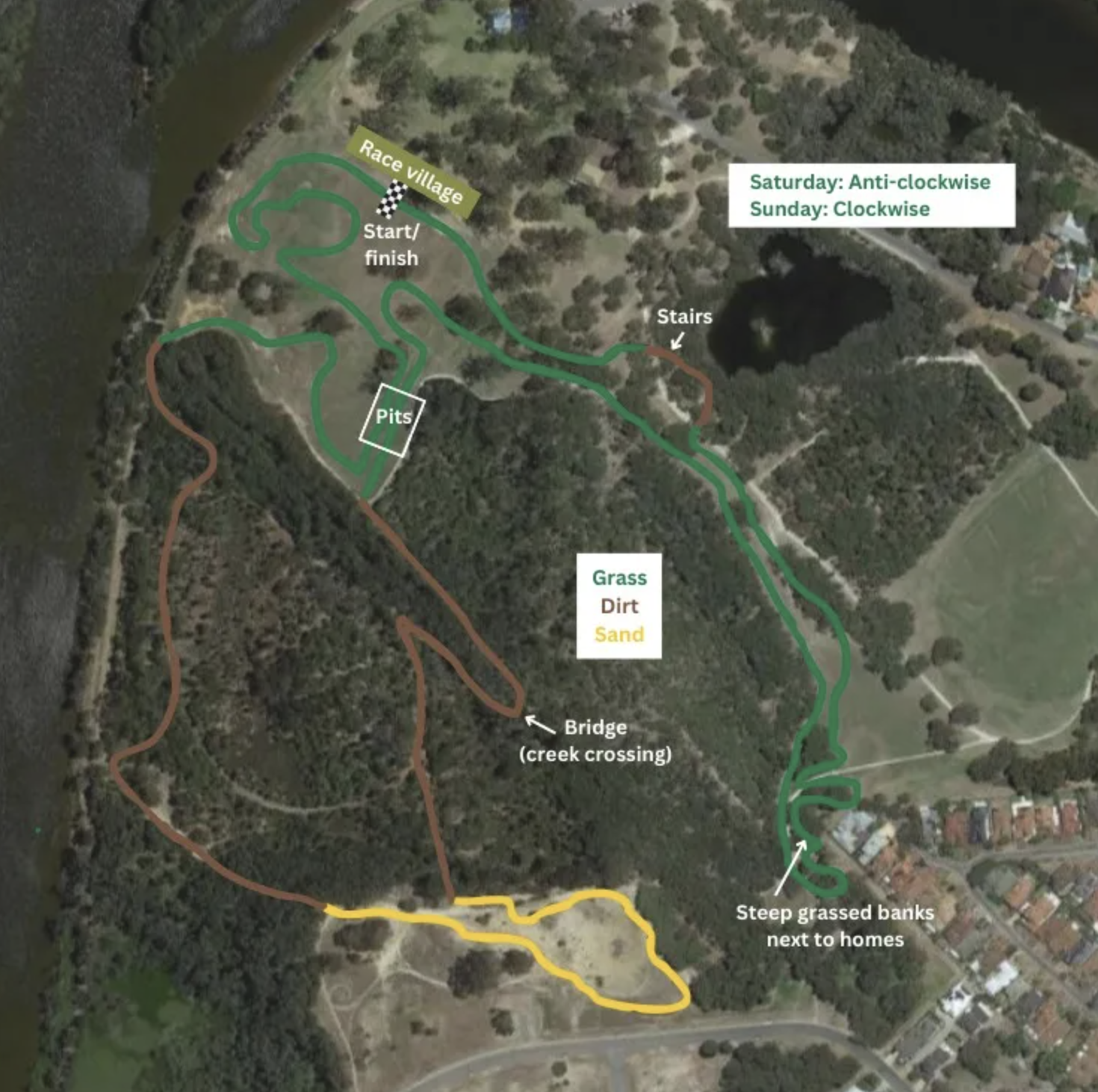This aerial map displays a detailed view of a wooded and residential area transformed into a racecourse. Dominated by various shades of green representing the terrain, the central focus is a zigzagging oval racecourse that traverses the middle of the image. At the top of the map, an olive green border marks the "Race Village" and the race’s "Start/Finish" line, complete with a small checkered flag icon. Below this, a white-lettered rectangle designates the "Pits."

Stretching throughout the map are colored lines, with green, brown, and yellow indicating different sections of the track—grass, dirt, and sand, respectively. These sections are detailed in a legend situated in the middle of the image. Labels are strategically placed on the map pointing out specific features, including "Bridge Creek Crossing" marked by an arrow to a brown area, "Steep Grass Banks next to homes" at the very bottom of the racecourse track, and "Stairs" indicating another notable section.

A small white border at the top right corner provides scheduling information, noting that races occur "Saturday: anti-clockwise" and "Sunday: clockwise." The overall landscape is interspersed with open areas among dense clusters of trees, adding to the complexity and challenge of the racecourse. The village housing development is conspicuously positioned to the very right of the photo, integrating residential elements with the racecourse layout.